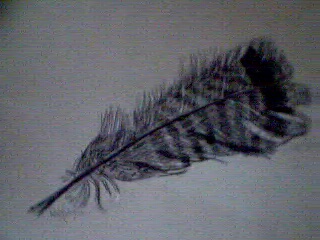In this image, a softly mottled dark gray background presents a subtly textured canvas, with darker hues particularly accentuating the edges. Dominating the scene is a striking feather that begins narrow at the base and expansively widens at the end. Its intricate coloring features a harmonious blend of gray, white, and black. The feather’s spine is distinctly black, providing a central anchor that runs longitudinally. Near the tips, a prominent black band encircles the feather just before transitioning into delicate light gray at the very edges. Throughout the feather, alternating stripes of light and dark gray add depth and contrast, interspersed with patches where black feathers intricately mingle within the pattern.